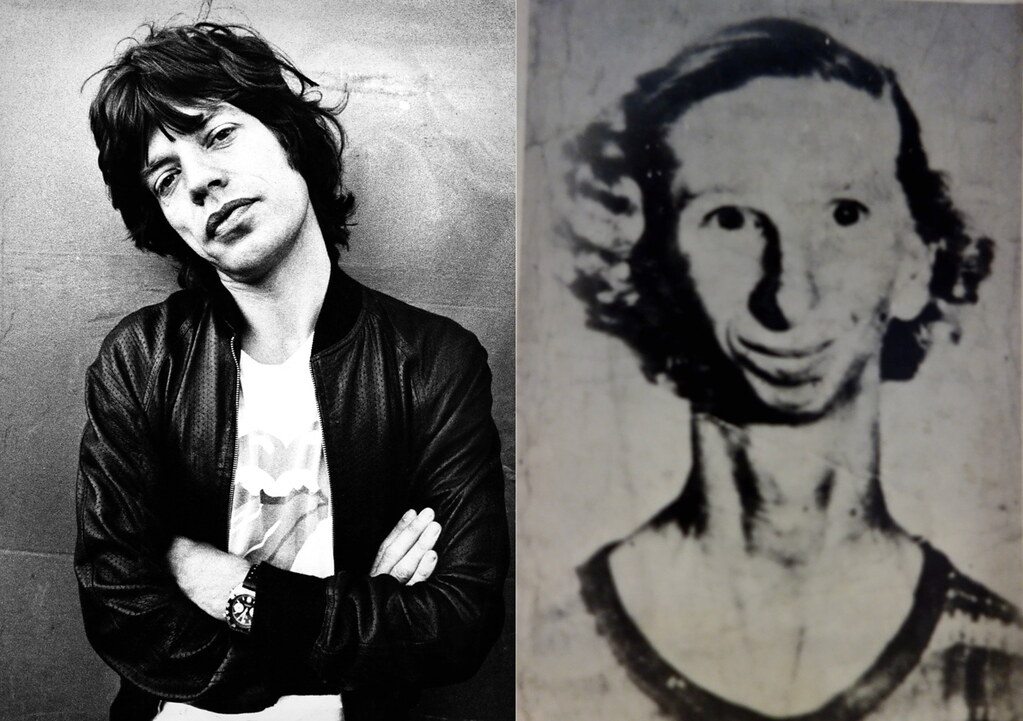The black-and-white photograph juxtaposes two distinct images. On the left is Mick Jagger, the renowned lead singer of the Rolling Stones, clad in a black leather jacket over a white t-shirt, with his dark scraggly brown hair framing his somewhat indifferent expression. His arms are folded in front of him, showcasing a wristwatch. On the right, an older and seemingly unrelated yearbook photo depicts a man with an abnormally long and thick neck, a small chin, wide eyes, and curly hair on the sides. The stark contrast between the widely recognized rock icon and the awkward, almost eerie appearance of the long-necked man draws attention, although the connection between the two remains unclear.